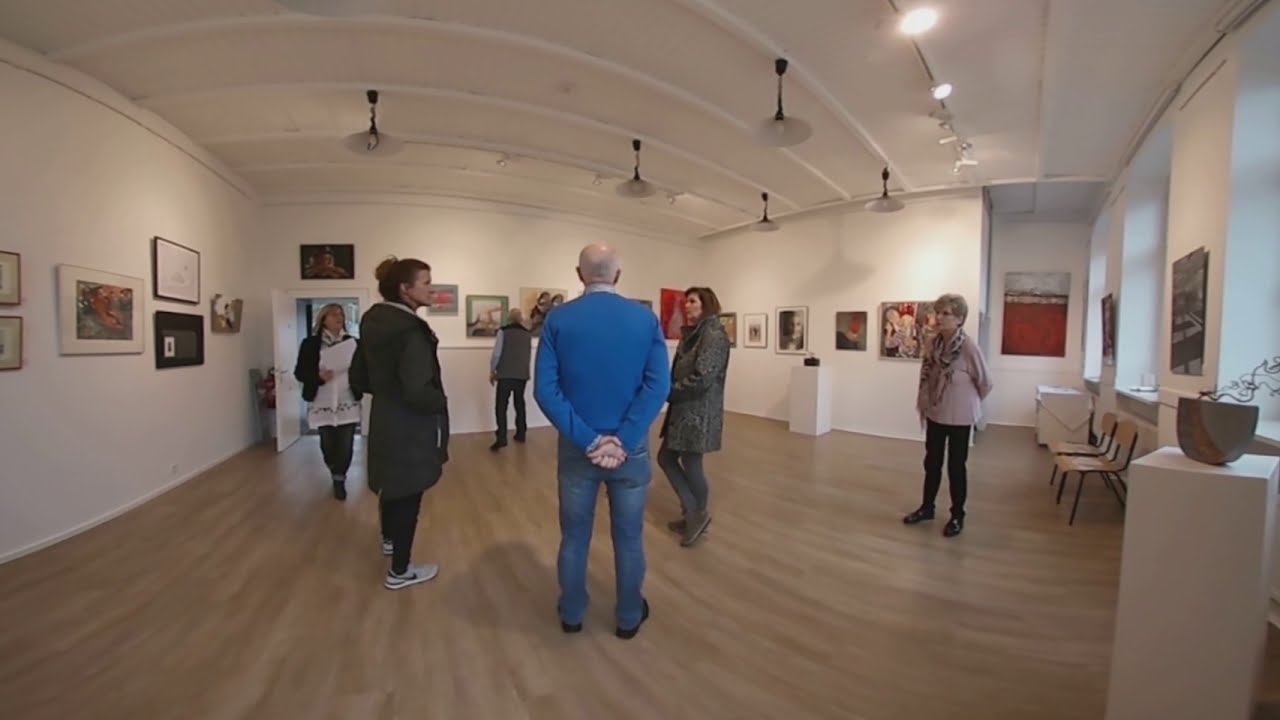In this detailed image, we observe a bustling art gallery with a tan pine hardwood floor. The expansive room has bright white walls adorned with framed paintings on all sides. The back wall curves slightly, adding architectural interest to the spacious environment, which is well-lit with overhead lights. Six older individuals, likely in their 60s and 70s, populate the scene, each absorbed in the surrounding artwork. 

At the center, a man with a blue jacket, blue jeans, and black shoes stands facing away from the camera, possibly engaged in a discussion about the art. To his left, a woman in a long gray hooded coat, wearing casual sneakers and black pants, takes in the paintings. Nearby, another woman in a tan outfit and black pants stands alongside two more individuals dressed in muted colors—gray, black, and white. One of these women is holding some paperwork, perhaps related to the gallery or the art. In the background, another man with a bald head and short gray hair on the sides, also in a blue long-sleeve sweater and denim pants, faces the back wall, deeply immersed in the artwork there.

The scene reveals both a serene and dynamic atmosphere, capturing the essence of art appreciation among the visitors in this dedicated painting room of the gallery.